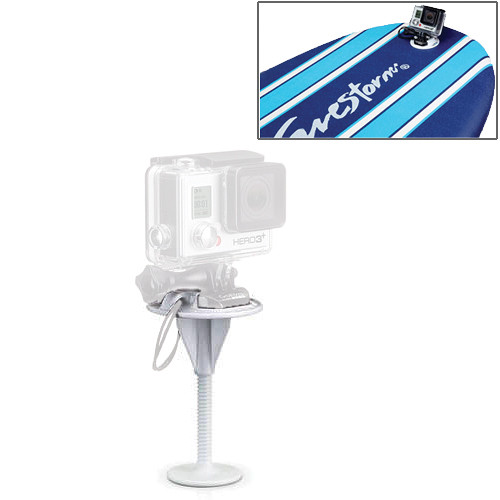This image showcases a Hero 3+ GoPro camera mounted on a surfboard using a specialized adapter. The surfboard, decorated with blue and light blue stripes, features the GoPro attached at the back end, facing the surfer. In the top right corner, a photograph highlights the surfboard setup, while the bottom left corner displays a close-up of the adapter, resembling a nail with a tripod top, designed to secure the GoPro to the surfboard with screws. The GoPro in the close-up is somewhat transparent and blurry, suggesting potential copyright constraints on the camera's image. The image is focused on demonstrating the practicality and design of the surfboard-mounted GoPro adapter.